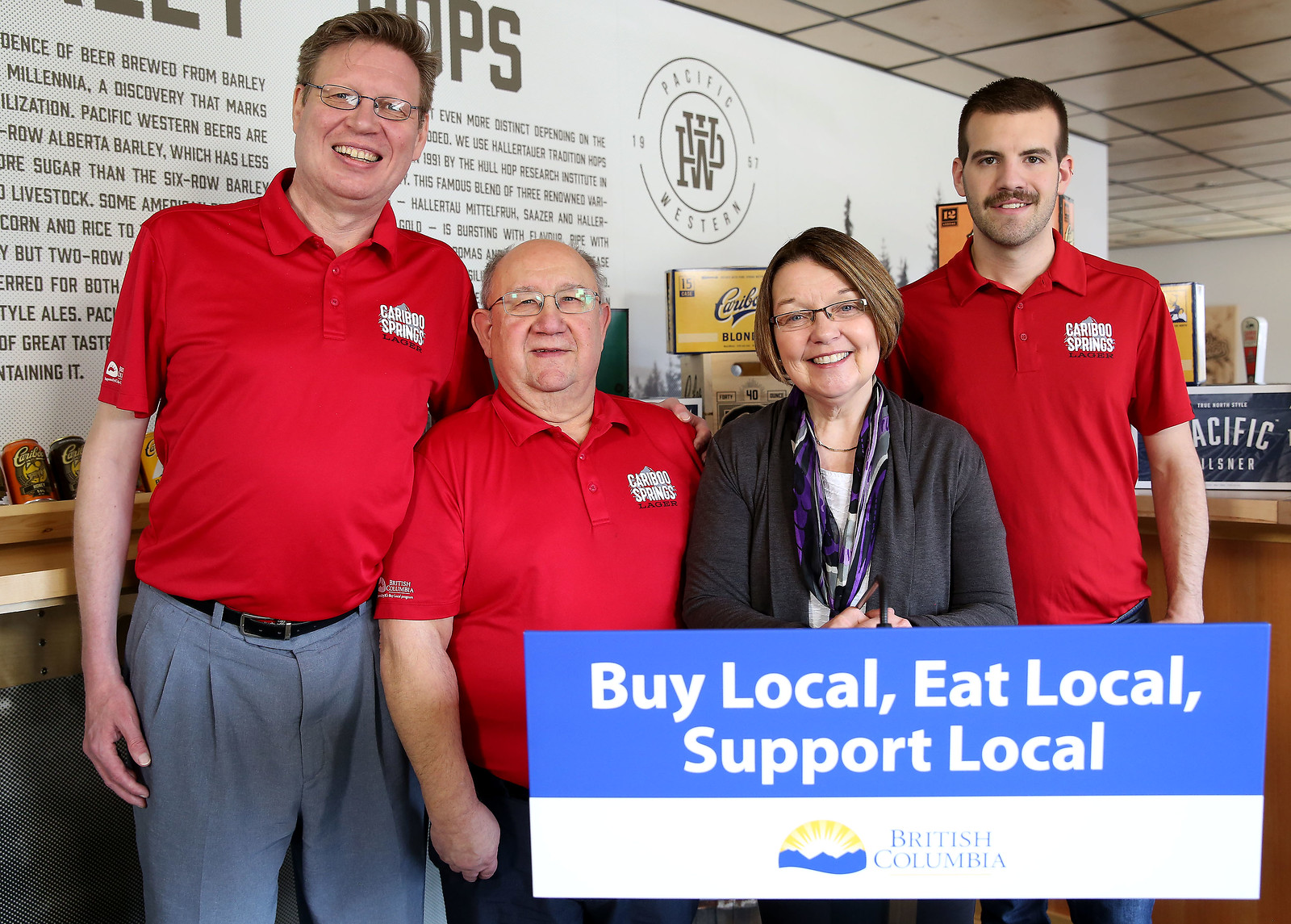The full-color photograph showcases an indoor promotional scene likely set in a restaurant or a brewery. It features four smiling adults: three men and one woman. The men, potentially representing three different generations—elderly, middle-aged, and mid-20s—are all dressed in identical red shirts emblazoned with "Caribou Springs Lager." The woman, distinguishable by her short brown hair, glasses, and outfit consisting of a white shirt, a gray jacket, and a purple scarf, offers a visual contrast. A prominent blue and white banner in front of them reads "Buy Local, Eat Local, Support Local," emphasizing its sponsorship by British Columbia. Additional details in the background include the name "Pacific Western" on the wall, pointing to the likely setting within a store or a similar commercial establishment. All participants exhibit a cheerful demeanor, reinforcing the supportive and engaging message of the local business campaign.